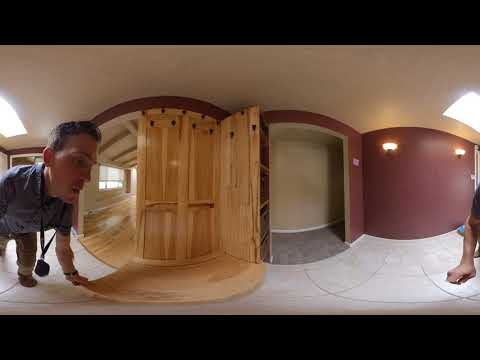The image features a distorted, surreal indoor scene bordered by thick black edges on the top and bottom. The photograph is in color, with no text. At the top, the ceiling is a tan color, featuring two lights, one on the far left and one on the far right. Below this, on the far left, a man wearing a blue shirt and some kind of object around his neck is depicted, looking to the right and slightly forward. He has short dark hair and a Romanesque facial profile. His presentation is highly distorted, with disproportionately small legs, a large head, and a small arm beneath him. He appears to be crawling or bent forward, possibly indicating he is working on a task, perhaps carpentry due to his posture and the tape measure-like object around his neck.

To the right of the man, the space is filled with wooden cabinets and a wooden floor, all similarly distorted. Further to the right, there is an archway leading into a gray-carpeted closet area. Immediately next, there’s a maroon-colored wall punctuated by two lights or sconces. On the right edge of the image, only an arm and a hand of another figure are visible, interacting with the white-tiled floor, potentially engaged in some task.

The perspective and image distortion create an unusual, almost surreal visual. Additionally, behind the man’s face, there appears to be a hallway with a window, and both the hallway and the room share a curved ceiling feature, amplifying the bizarre and strangely patterned appearance of the scene. The scene is brightly lit, although the type of room remains ambiguous, possibly suggesting a hallway or a changing room.